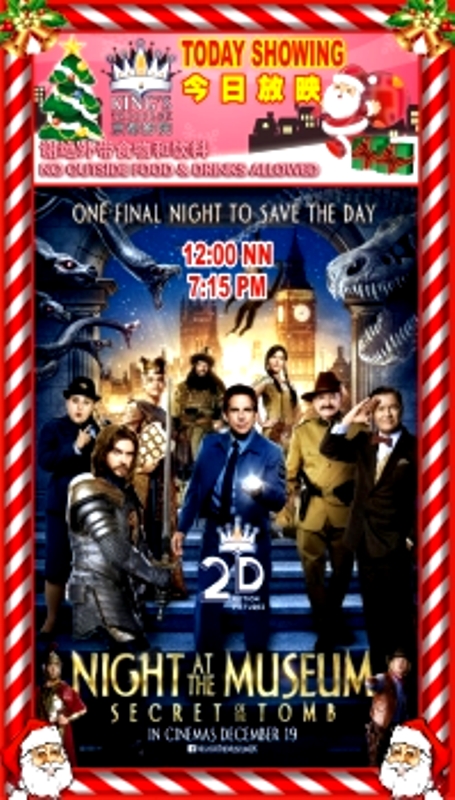This vividly detailed image features a movie poster for "Night at the Museum: Secret of the Tomb," framed with a festive, candy-cane striped border. The top corners of the frame are adorned with golden bells and holly, while the bottom corners showcase Santa Claus heads complete with white beards and hats.

At the very top of the poster, a bold red banner exclaims "Today's Showing" along with a warning against bringing outside food and drinks. Beneath this, there are some Chinese characters, enhancing the international festive feel. Also featured on the top section are a crown, a cartoon Santa Claus, and multiple Christmas trees in the bottom corners.

The central portion of the poster prominently displays the movie's title, "Night at the Museum: Secret of the Tomb," indicating a release date of December 19th and noting the film is available in 2D. The tagline, “One Final Night to Save the Day,” stretches across the top of this central image. The characters of the movie, including Ben Stiller and Robin Williams, along with elements like dinosaurs and notable landmarks such as Big Ben, add to the visual intrigue. Additional details include a group photo of the characters, a T-Rex skeleton, and some snakes, providing a glimpse into the adventurous and whimsical nature of the film.